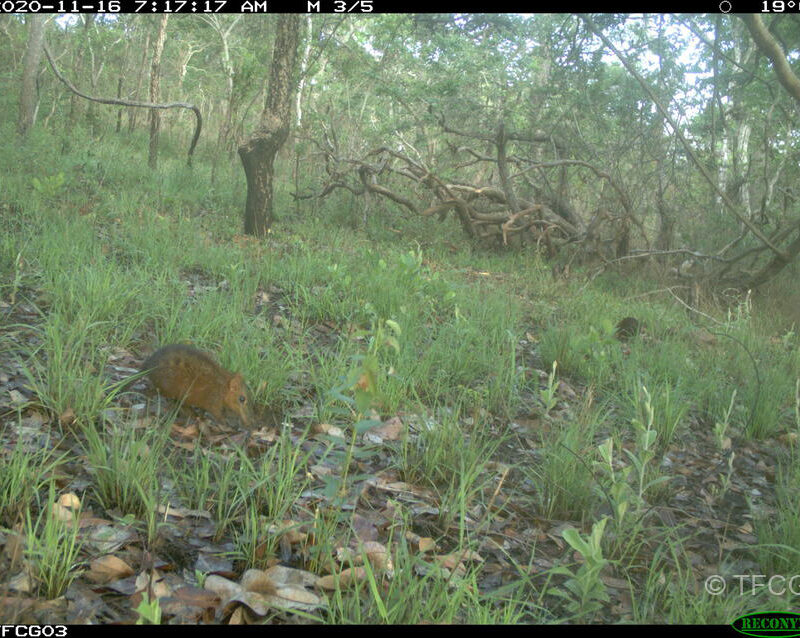The photo appears to be a still from a surveillance camera positioned in a woodland area. In the foreground, a small brown rodent, possibly a rat or another species of rodent, is captured. The rodent features dark eyes and a long nose and roams among patches of grass that are tall but not overly dense, allowing a clear view of the animal. The woodland setting includes a mix of standing and fallen trees, some of which have unusual growth patterns, curving horizontally before continuing upward. The background shows both logs and dry trees that have fallen, adding to the rugged, natural atmosphere. The date, time, and temperature are displayed in a black bar at the top of the image, indicating that it was taken on November 16, 2020, at 7 a.m. with a temperature reading of 19 degrees.